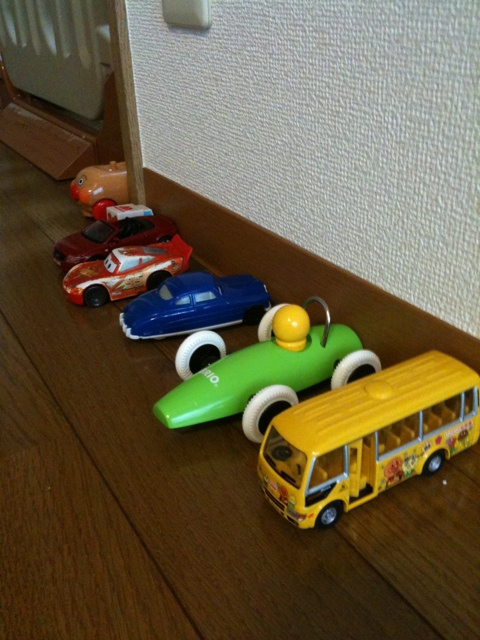The photograph captures a scene within a house, showcasing a vertical orientation that emphasizes the height of the room over its width. The room features dark wooden floors and a matching dark brown baseboard, grounding a textured off-white wall adorned with a distinctive pop-out grid pattern. Arranged meticulously along the baseboard are six vibrant children's toy vehicles, poised as if ready for a race. Starting from the left, a brown car with cheerful orange wheels and a face leads the lineup. Next to it is a dark red car, followed by a character car from the Disney Cars movie with two expressive eyes on the windshield, resembling Lightning McQueen. Continuing the lineup, there is a blue classic car with white details, a green race car, and a yellow school bus. Despite a couple of the toys facing the opposite direction, the arrangement retains a playful and nostalgic ambiance, reminiscent of childhood days. The orderly presentation against the contrasted wooden floor and textured wall highlights the simple yet creative staging of the image.